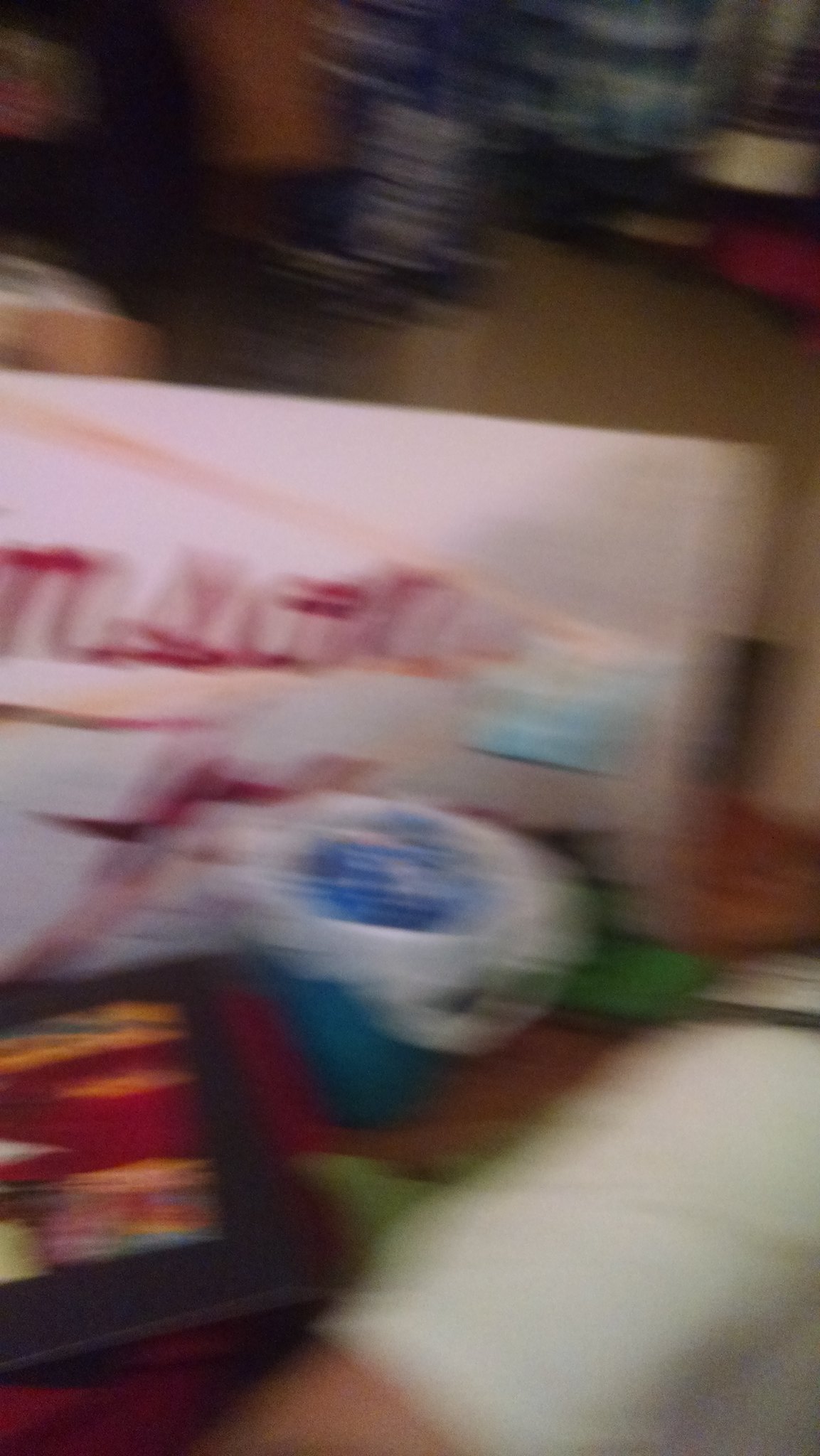This image is very blurry, obscuring much of the detail, but it seems to depict a domestic setting. At the center of the image, there is a white rectangular object resembling an envelope or poster board with red writing on it, possibly handwritten with a marker. This object is notably blurred, making the writing indistinguishable. Positioned in front of this is a small blue trash can or tub, approximately half the height of the white rectangle, featuring a white liner with visible contents inside. 

To the lower right of the image, there is a Caucasian arm, seemingly belonging to someone wearing a t-shirt, extending from the right side and exiting towards the bottom left. Also, on the lower right-hand corner, there's an item resembling either a white towel or shoebox. In the background towards the top, there appears to be a closet with hanging items. The setting suggests that the objects might be placed on a couch, chair, or possibly the floor of a room. Additional items like a colorful object, perhaps an iPad, and some wooden structure, possibly part of a piece of furniture, are also seen within the blurry image, adding to the cluttered yet domestic aura of the scene.